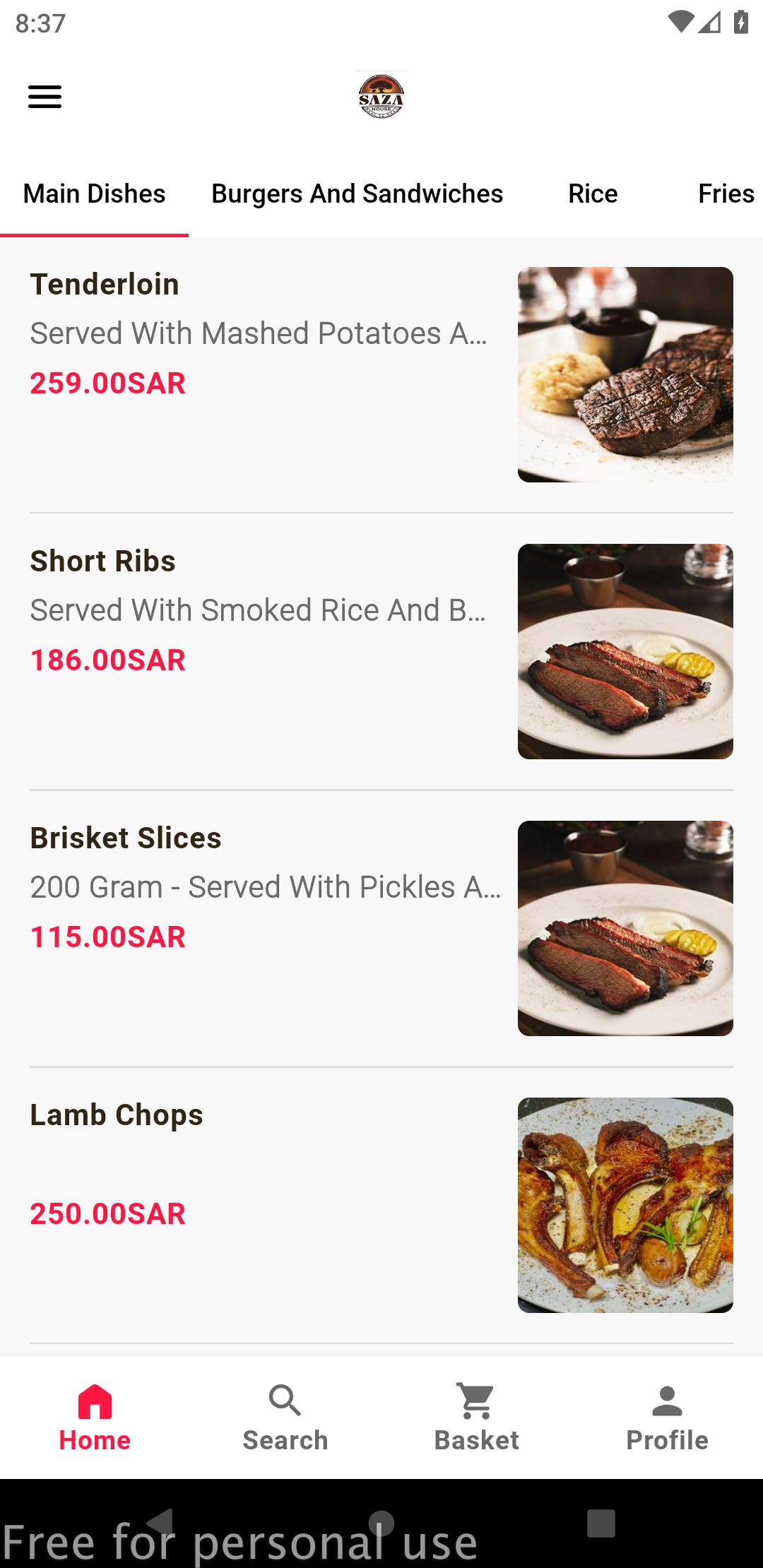**Detailed Caption:**

This is a detailed screenshot of a restaurant's web page taken at 8:37 AM, as indicated by the device's clock in the upper right corner. Alongside the clock, there are icons displaying the internet connectivity and phone battery charge. On the upper left, there is a menu represented by three horizontal bars. At the very top, there is a small, round icon with indistinct text that seems to read "K-A-Z-A."

Beneath the top navigation bar, the page showcases four main categories: "Main Dishes," "Burgers and Sandwiches," "Rice," and "Fries." The "Main Dishes" category is currently highlighted, suggesting it is the active selection.

Displayed prominently are four menu options under the "Main Dishes" category. 

1. **Tenderloin Served with Mashed Potatoes:** 
   - Price: 259.00 SAR
   - A picture to the right shows a neatly charred tenderloin steak on a white plate, accompanied by a side of mashed potatoes and a small cup containing an unspecified item.

2. **Short Ribs Served with Smoked Rice and Be...:**
   - Price: 186.00 SAR
   - The image depicts what appears to be a misrepresented dish. Although labeled as short ribs, the picture actually shows sliced brisket fillets, possibly filet mignon, with a lemon slice on a white plate.

3. **Brisket Slices - 200 grams Served with Pickles:**
   - Price: 115.00 SAR
   - The picture mirrors the one used for the short ribs, signifying an error. Both show the same brisket slices with a lemon slice.

4. **Lamb Chops:**
   - Price: 250.00 SAR
   - To the right is a plate showcasing short ribs (though listed as lamb chops), served with vegetables and a side of rice.

At the bottom, the page has a navigation bar featuring four icons: "Home," "Search," "Basket," and "Profile," allowing users to easily navigate through the website.

This screenshot summarizes a snapshot of the restaurant's digital menu, highlighting both visual and text elements, though it makes note of inconsistencies between the food descriptions and their images.